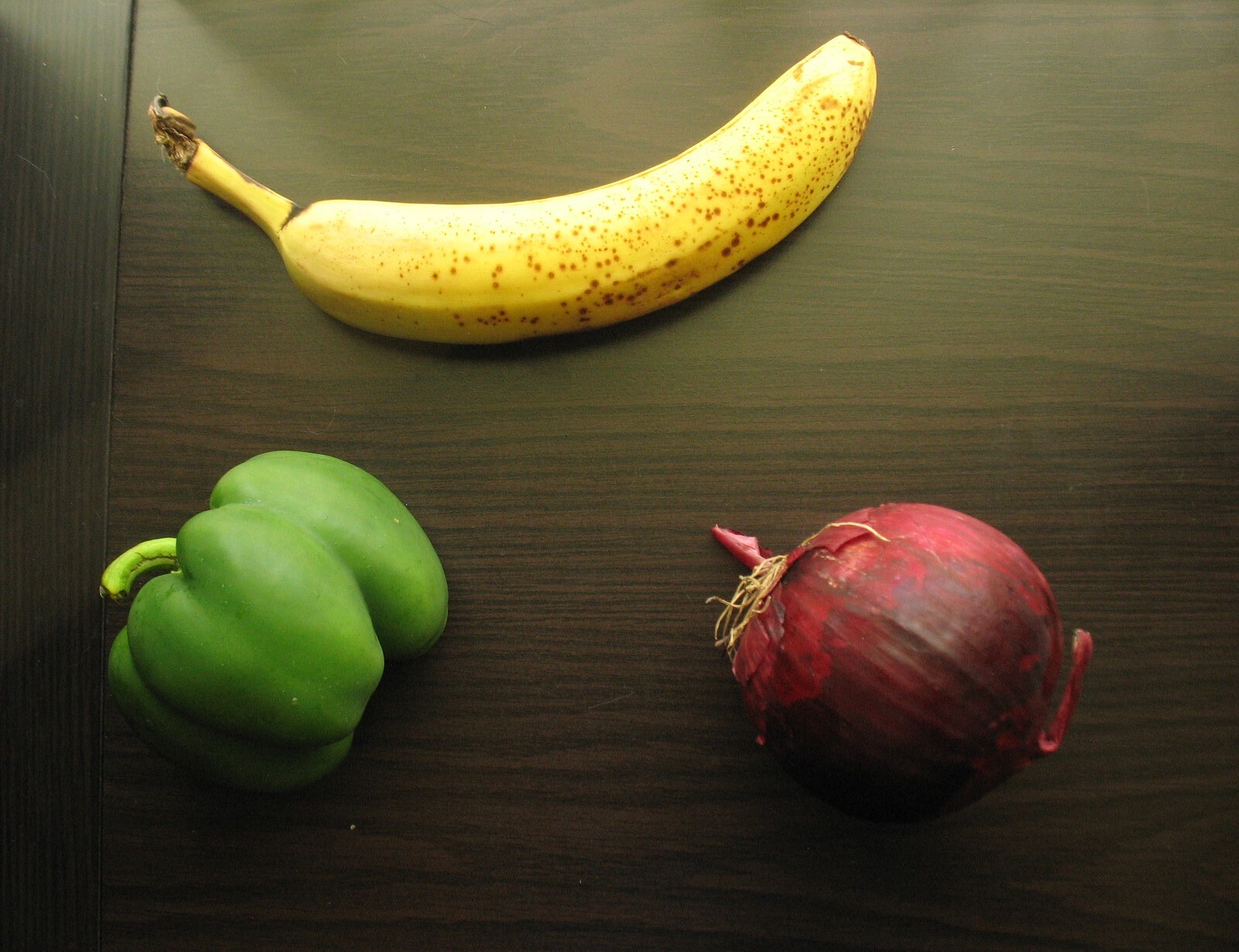A close-up image showcases a variety of fruits and vegetables artfully arranged on a vintage brown vinyl table. Prominently placed at the top center is a perfectly ripe banana, noted for its vibrant yellow color accented with a few brown spots, indicating optimum ripeness. To the left-hand corner, a luscious and healthy yellow bell pepper stands out with its bright hue and full, round shape. The bottom right corner features a robust red onion, exhibiting minor stippling on its skin, suggesting that the outer layers might need to be peeled to reveal its fresh interior. The table, though old in appearance, is clean and adds a rustic charm to the composition. A light source from above bathes the banana in a gentle glow, highlighting its readiness to be enjoyed. This picture captures the natural beauty and varying stages of freshness of these everyday produce items.